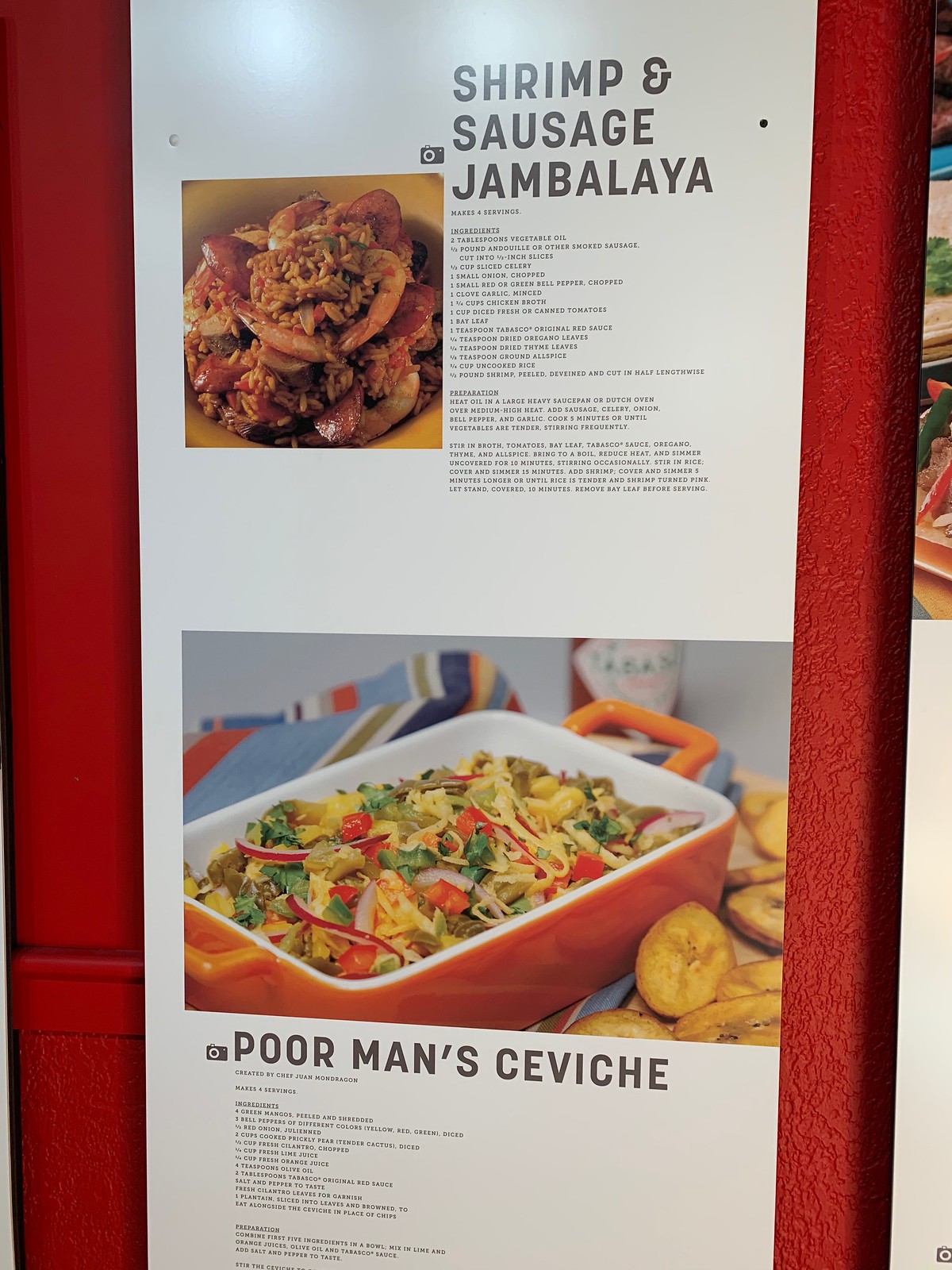In front of a red wall, there is a tall sign, possibly made of cardboard or wood, featuring two large white recipe cards stacked vertically. The top card showcases a vibrant photograph of shrimp and sausage jambalaya in a yellow bowl, accompanied by small, illegible black text presumed to be the recipe. Below it, a space of white separates this from another photograph displaying 'poor man's ceviche' in an orange and white casserole dish, surrounded by plantains atop a blue multi-colored striped tablecloth with a bottle of Tabasco sauce in the background. The text beneath this image is also too small to read fully, and the bottom part of the recipe is cut off in the image. Both cards appear to be part of a menu or a display in a restaurant, emphasizing the specific dishes with visual and textual detail.